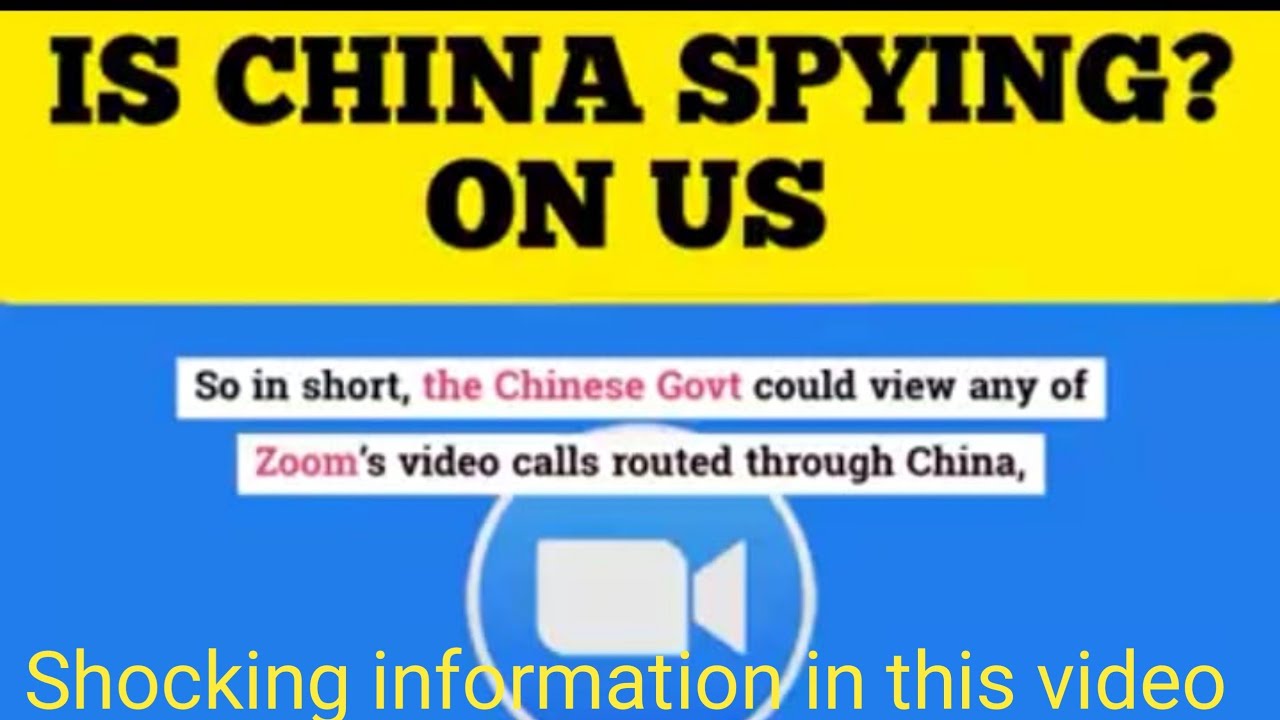The image is split into two halves with the upper portion featuring a solid yellow background and the lower half a blue background. At the top of the yellow section, a thin black border spans horizontally. Centered prominently in this area, bold black letters pose the question: "Is China spying on us?"

On the blue bottom half of the image, two white text boxes provide further insights. The first text box, located towards the top of the blue section, reads: "So in short," followed by "the Chinese Govt," with "Govt" abbreviated in bold red letters and the initial "G" capitalized. Continuing in black ink, it states: "could view any of."

The second text box, located below the first, declares in bold red font, "Zoom's" with the apostrophe "S" in black ink, followed by black text that reads, "video calls routed through China."

In the background of the blue section, centrally positioned, is an icon of a video camera inside a white circle. Overlaying the image towards the bottom foreground, bold yellow letters convey a notable message: "Shocking information in this video."